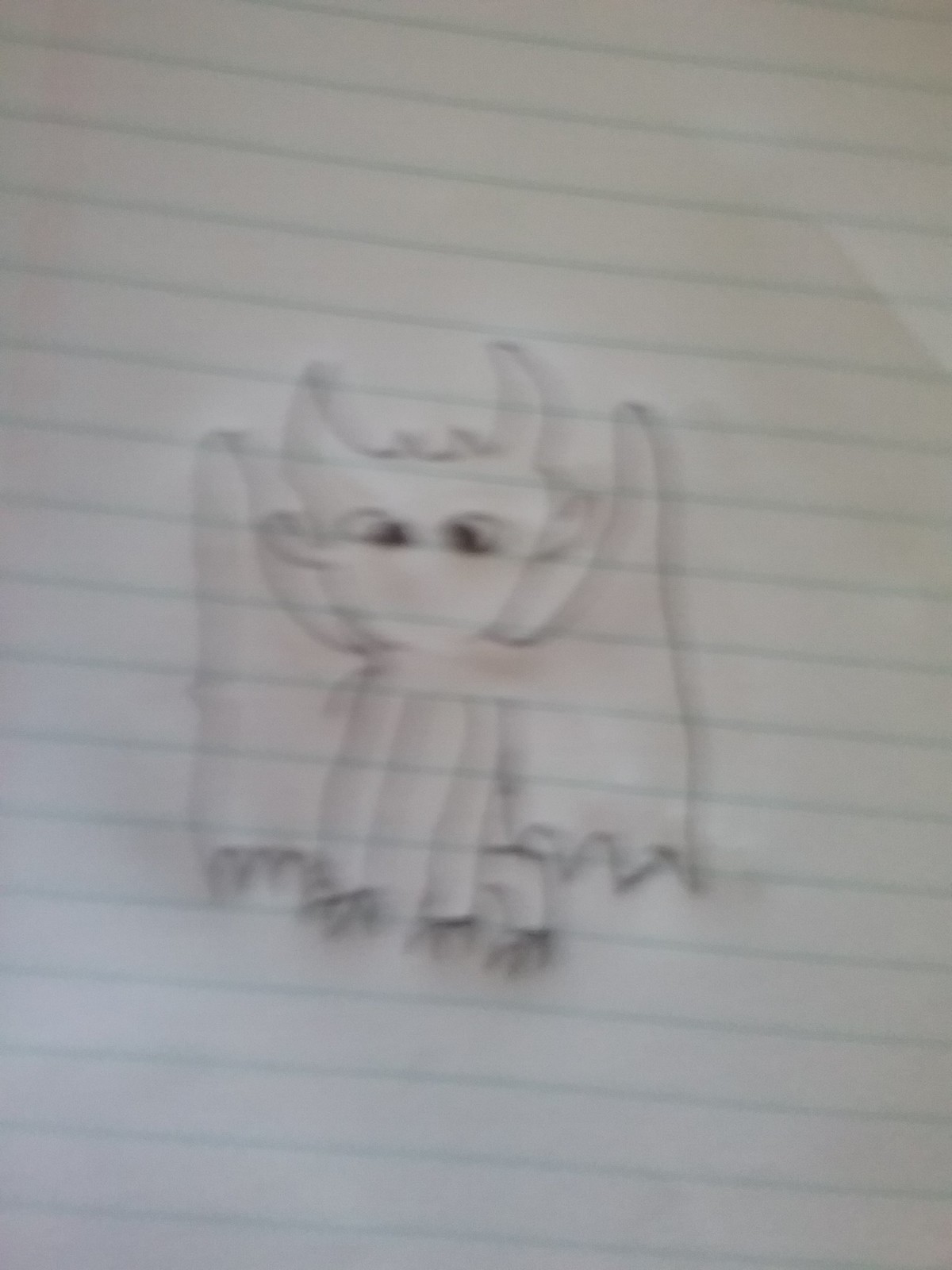The image is a rectangular, blurry photograph of a basic pencil or pen drawing on a piece of notebook paper. The notebook paper has light green lines that are slightly diagonal, running from the bottom right towards the top left corner. The drawing, done in dark pencil or pen, depicts a small winged creature situated in the center of the page. This creature has prominent, bat-like wings emerging from its back, and its body comprises two long front legs and two back legs, each terminating in three claws. The head, which is relatively large in proportion to the body, features two large human-like eyes and two upward-curving horns. The creature's overall appearance combines bat-like and cat-like characteristics, making it resemble a bat with a cat-shaped head and long limbs. Despite the sketch's blurred quality and the slight angle at which the photograph was taken, the unique details of the winged monster—the horns, claws, and sizable wings—are discernible, suggesting a fantastical or imaginative creation, potentially drawn by a child.